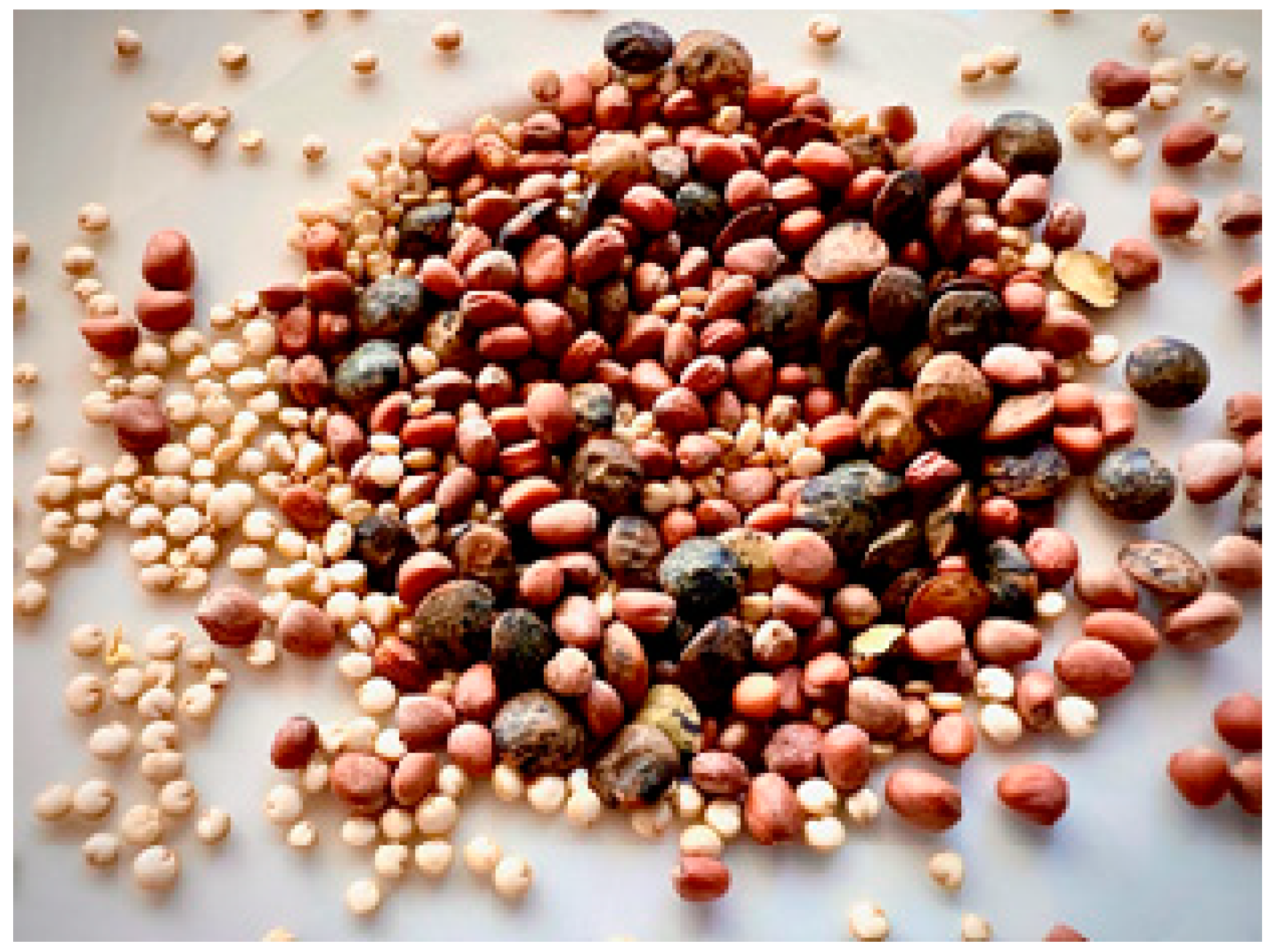This is a very pixelated and unclear close-up image showing an assortment of grains, beans, and possibly nuts or legumes splayed out on a white surface, which might be a table or countertop. The image quality is poor, with visible square pixel shapes and stitching lines that indicate it has been stitched together from multiple pictures. The items appear to vary in size and color, including small, light tan, and larger, darker brown beans, as well as round, speckled beans with a mix of dark and light brown. Some objects resemble small pinto beans, lentils, or dried corn. The grains and legumes are densely piled in the center, becoming more loosely spread out toward the edges. The entire composition is blurry and difficult to decipher with precision.